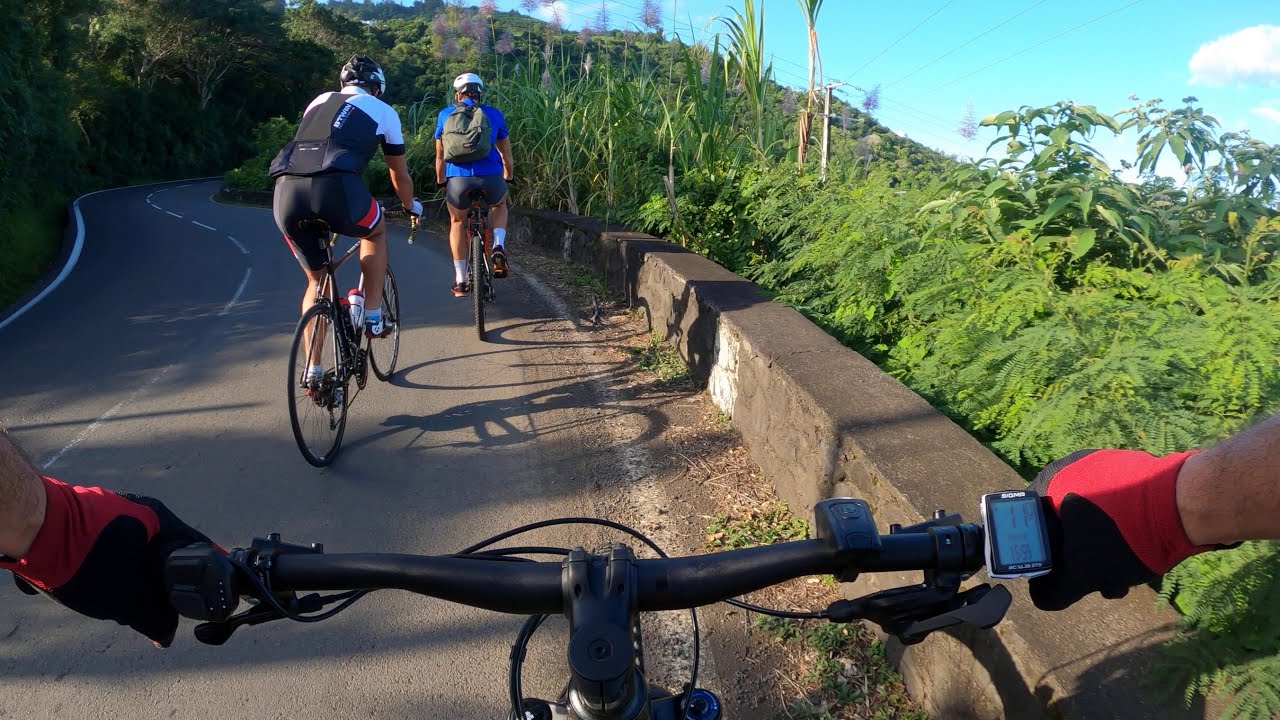The image captures a first-person view from a cyclist riding up a hill on a paved road, possibly during a biking race or a casual ride. The cyclist's hands, clad in red and black gloves, firmly grip the left and right handlebars of their bike. A small device displaying numerical data, possibly a trip meter or distance tracker, is mounted on the right handlebar, showing figures such as 11 and 15:59. Another device is visible near their left hand. In front of this cyclist, two other bicyclists, dressed in distinct cycling gear—one in a blue shirt with black shorts and the other in an outfit of black, white, and red—ride up the hill. The road, devoid of any vehicles or pedestrians, is flanked by a concrete slab on the right side, separating it from an area covered in trees and bushes. Additional vegetation lines the left side of the street. The clear quality of the image, taken during the daytime, showcases a bright blue sky with white clouds, highlighting the desolate yet scenic route the cyclists are traversing.